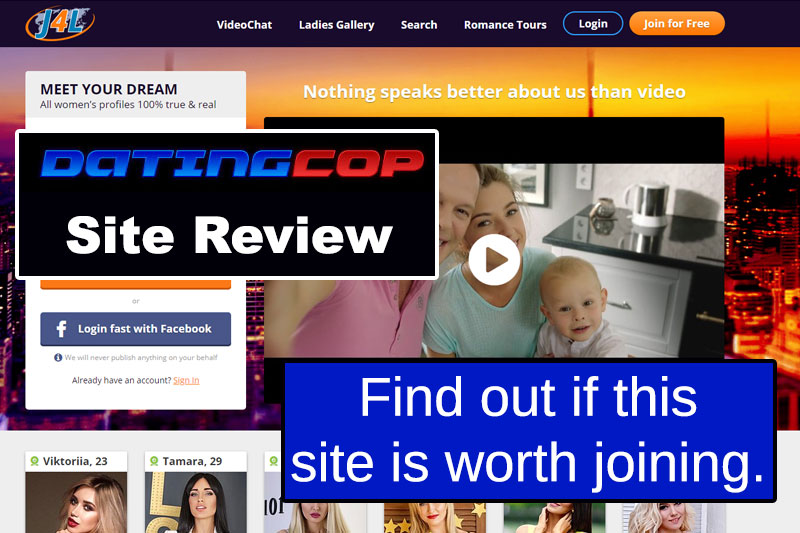This is a screenshot of a dating website featuring a sleek and modern design. The top banner is a striking dark blue mixed with purple tones. In the upper left-hand corner, the site's logo is prominently displayed: the letters "J4L" with the "J" and "L" in blue and the "4" in orange. This logo is set against a world map backdrop, encircled by an orange halo.

At the very top of the page, there are various navigation options for users, including "Video Chat," "Ladies Gallery," "Search," and "Romance Tours." There are also buttons for "Login" and "Join for Free." Directly beneath this navigation bar, an eye-catching tagline reads: "Nothing speaks better about us than video."

Highlighted prominently below the tagline is a large video player with a play button at the center. The freeze-frame depicts a man, a woman, and a baby in a kitchen setting. Adjacent to the video, bold text declares: "Meet your dream. All women's profiles 100% true and real."

Overlaying the entire image are two large text boxes. The one on the left reads: "Dating Site Review," and the one below it prompts users to "Find out if this site is worth joining."

Finally, at the bottom of the screenshot, there is a gallery of women's pictures, each accompanied by their names and ages, inviting users to explore potential matches.